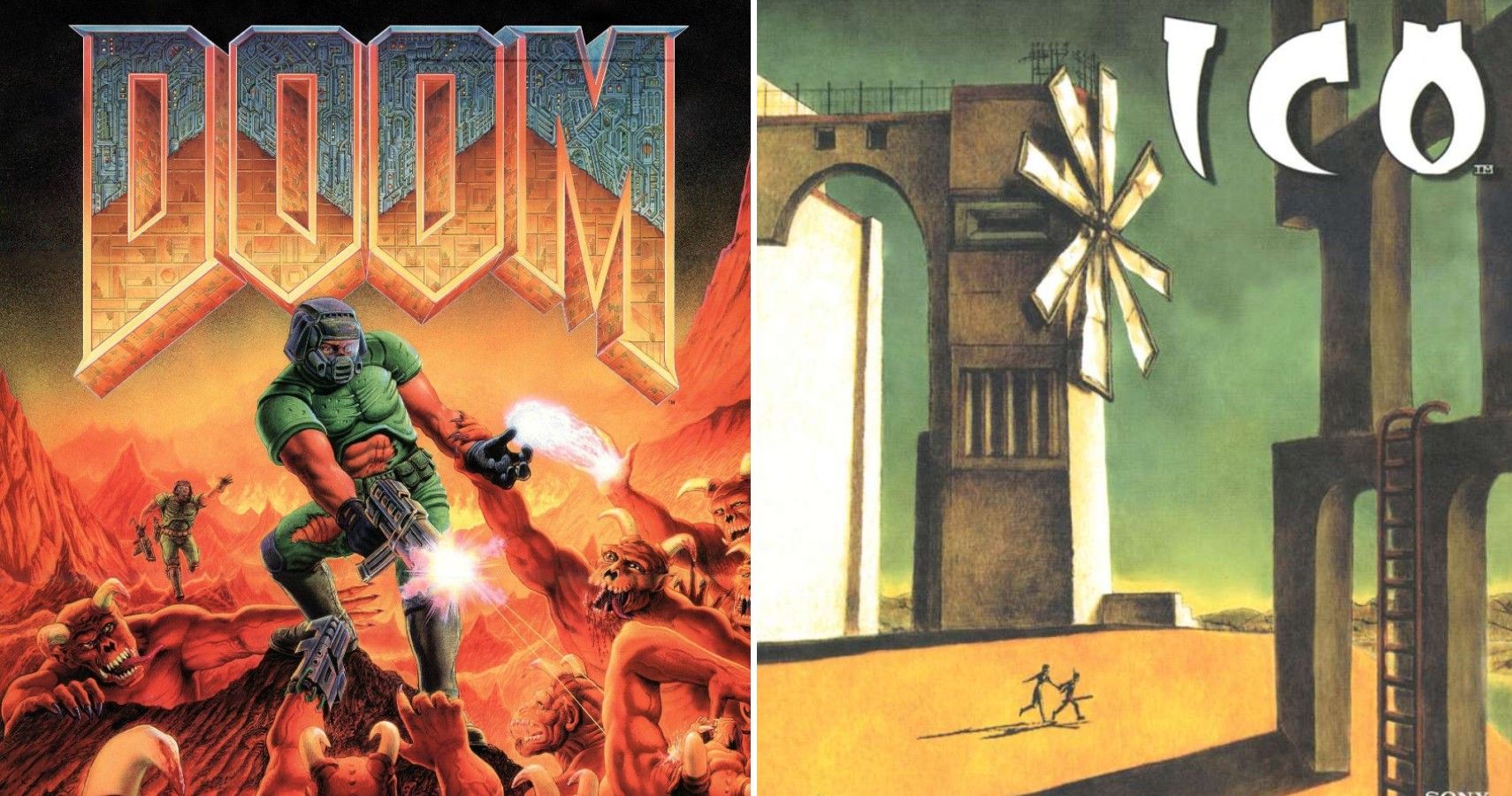This combined image consists of two distinct panels, each resembling the cover art for video games or digital artwork. 

The panel on the left prominently features the title "DOOM" at the top. It depicts a dramatic and intense scene in which a man, clad in a green combat suit and military-style helmet, is standing heroically with one leg propped on a rock. He wields guns in both hands, aiming downwards at monstrous creatures below. These creatures have menacing horns and their tongues protruding out, appearing aggressive and threatening. In the background, another figure dressed similarly in a green suit is seen running towards the central character with an arm raised, seemingly attempting to warn or signal him.

The panel on the right offers a stark contrast with a calmer, green-hued background. It features a building with an unusual windmill structure. The title "ICO" is imprinted on the front. In the foreground, two small human figures are visible, dwarfed by the architecture. The building appears to have several doorways but lacks other visible structural elements, giving it an abstract appearance. A ladder extends to one of the doorways, adding to the enigmatic and tranquil vibe of this part of the image.